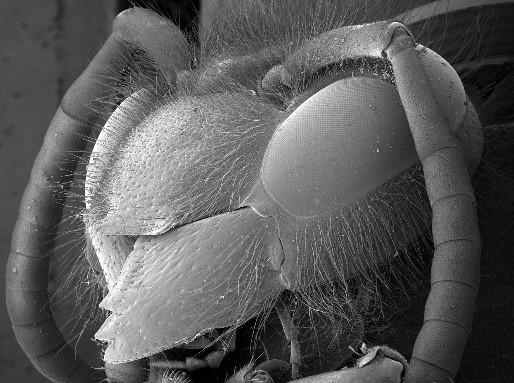This is an intricately detailed, monochromatic gray, microscopic view of an insect's head, likely that of an ant or a fly. The high-resolution image shows the insect’s head adorned with numerous hair fibers that extend around and on top of the head. Prominent antennae extend from the top of the head, wrapping down along the sides. Each antenna features transverse lines and falls alongside the head. The insect’s eyes, positioned on either side of the head, resemble a grid pattern, indicative of their compound structure. Additionally, a sharp, central nose-like feature can be observed. The entire image is rendered in black and white, enhancing the clarity of the fine details such as the multitude of tiny hairs covering the insect’s face, contributing to the overall fuzzy appearance.